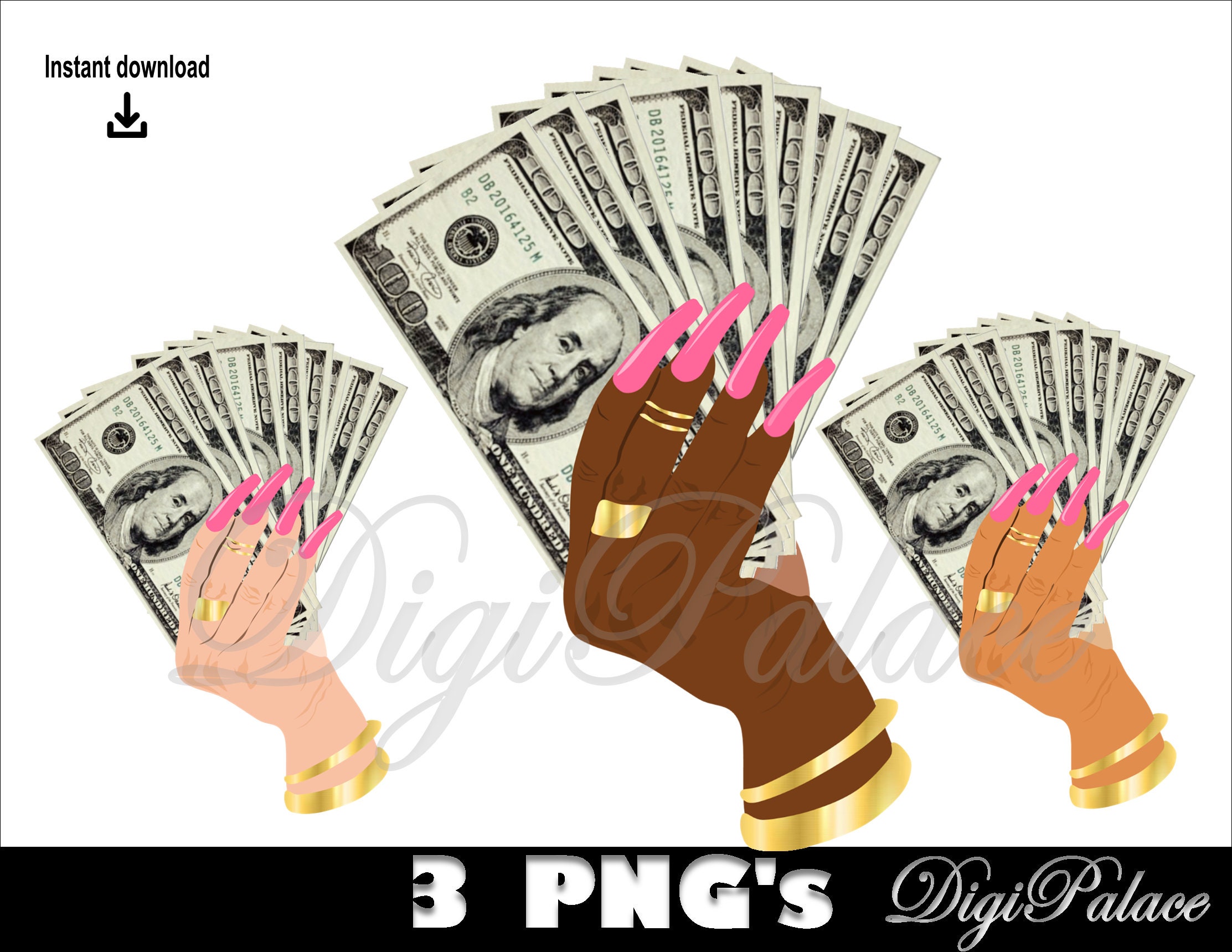The image is an advertisement featuring three women's hands with long pink nail extensions, each holding a fan of $100 bills. The background is mostly white, especially in the upper left corner where an "instant download" icon is displayed, showing a tray with a downward arrow. At the bottom, a narrow black banner with white text reads, "three PNGs DigiPalace." The hands vary in skin tone: the left hand is Caucasian, the center hand is African American, and the right hand has lighter brown skin. All hands are adorned with gold rings and bracelets. The overall aesthetic of the image hints that it might be computer-generated rather than an actual photograph. The text at the bottom and the overall layout suggest it is promoting downloadable PNG files, likely for digital art or graphic design purposes.